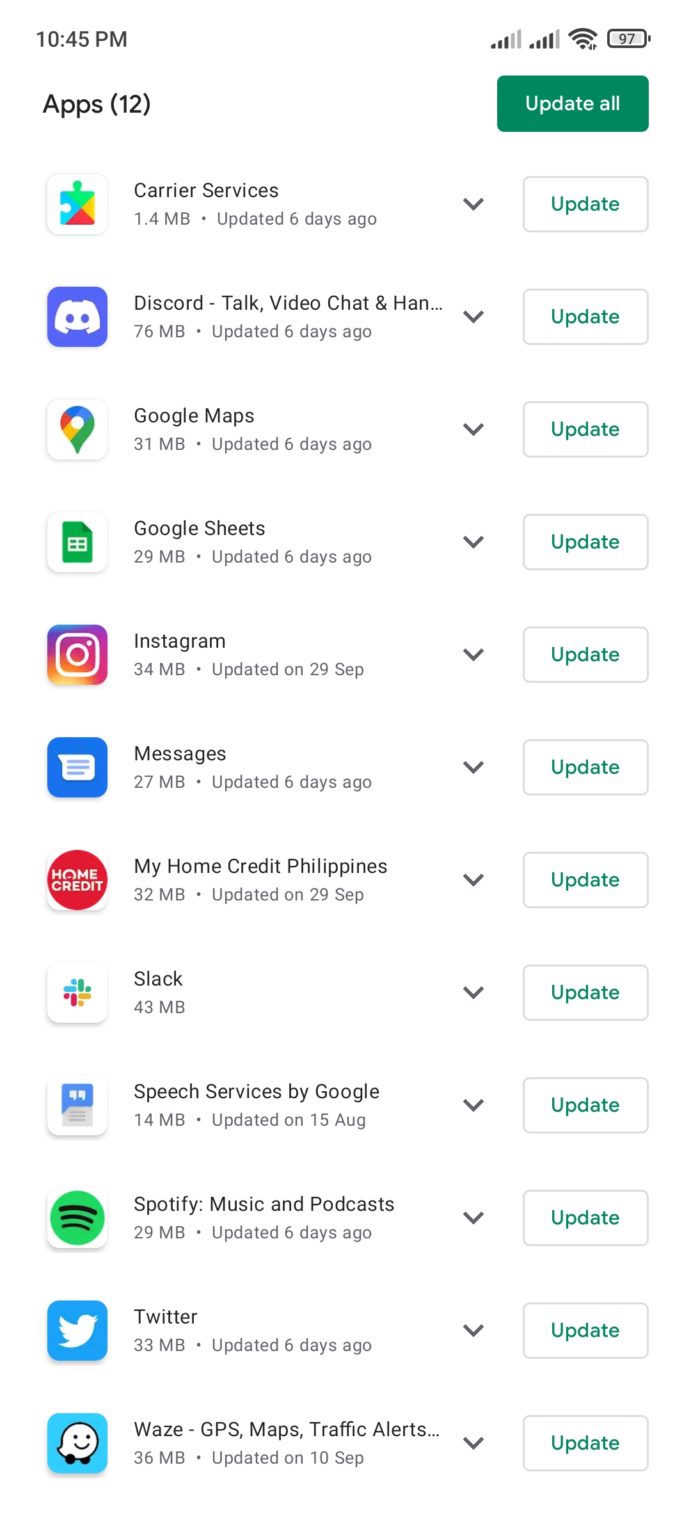The image is a screenshot from what appears to be the App Store or a similar app library interface. At the very top left of the screen, the time displayed is 10:45 p.m. On the top right, there are icons indicating two data bars, Wi-Fi connectivity, and a battery icon showing 97% charge. Below these icons, a prominent green button labeled "Update All" is situated. To its left, the word "Apps" is displayed followed by the number 12 in parentheses, indicating the total number of apps.

The list of apps awaiting updates includes:

1. Carrier Services
2. Discord
3. Google Maps
4. Google Sheets
5. Instagram
6. Messages
7. My Home Credit Philippines
8. Slack
9. Speech Services by Google
10. Spotify
11. Twitter
12. Waze